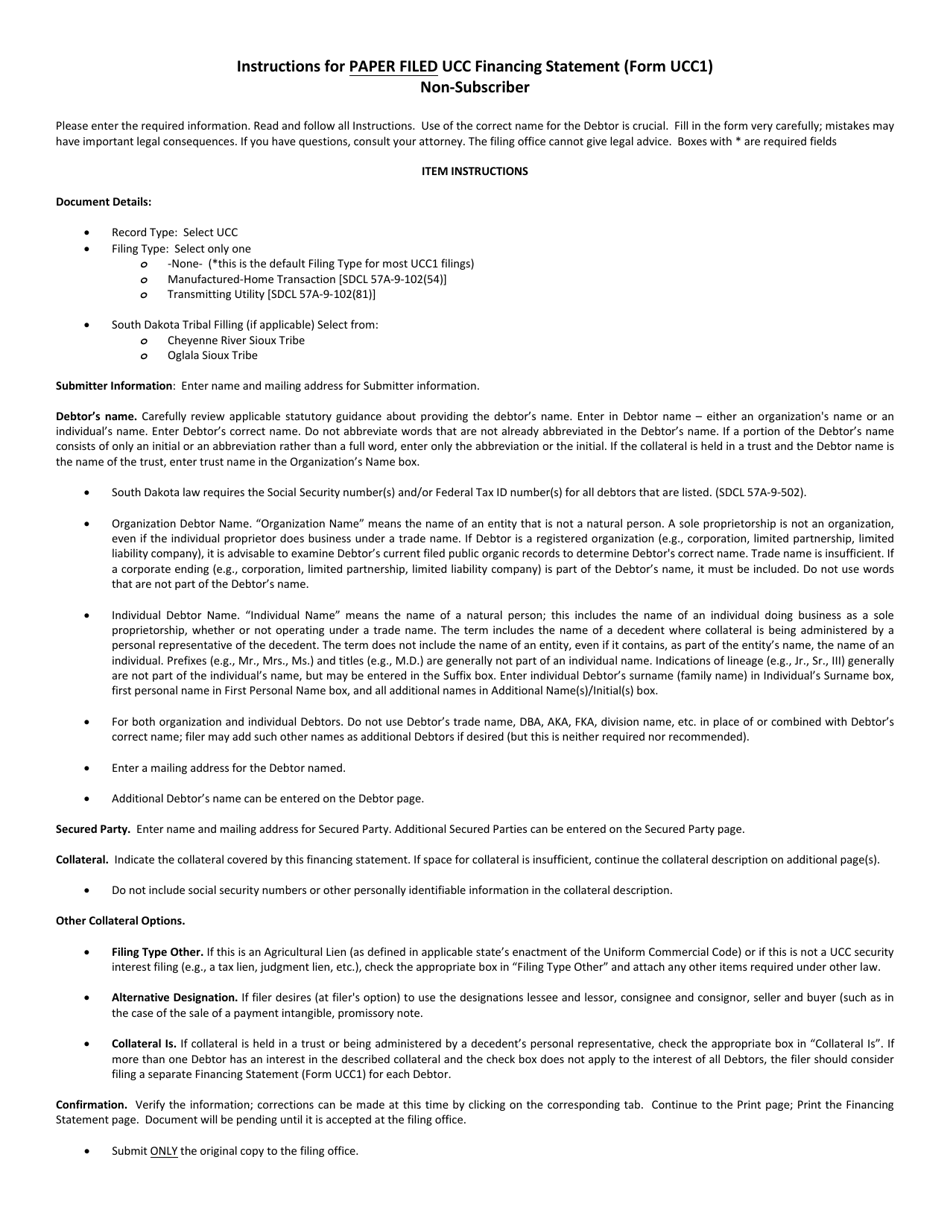This screenshot captures a document titled "Instructions for Paper-Filed UCC Financing Systems (Form UCC-1)." The title, prominently displayed in black at the center top, is underlined and followed by "non-subscriber paper file."

The document begins with several key instructions:

- "Please enter the required information."
- "Read and follow all directions."
- "Use of the correct name for the debtor is crucial."
- "Fill in the form very carefully."
- "Mistakes may have important legal consequences."
- "If you have questions, consult your attorney."
- "The filing office cannot give legal advice."
- "Boxes with an asterisk are required fields."

Next, there is a section titled "Item Instructions," under which "Document Details" are provided. The details include:

- **Filing Type:** "South Dakota Tribal Filing Select Form"
  - **Two Tribes Listed:** Cheyenne River Shooks Tribe and Olalla Tribe

Additionally, there are fields for:

- **Submitter's Information:** Includes the name and mailing address of the submitter.
- **Debtor's Name**
- **Secured Party**
- **Collateral Options:** Which encompass "filing other type," "alternative designation," and the specific "collateral."

The final section, "Confirmation," emphasizes the importance of verifying all entered information. It instructs to "verify the information" and explicitly states, “submit only the original copy to the filing office,” with "only" being underlined for emphasis.

This detailed caption encapsulates the structure and critical aspects of the document, guiding users on the precise and careful completion of Form UCC-1 for paper filing.